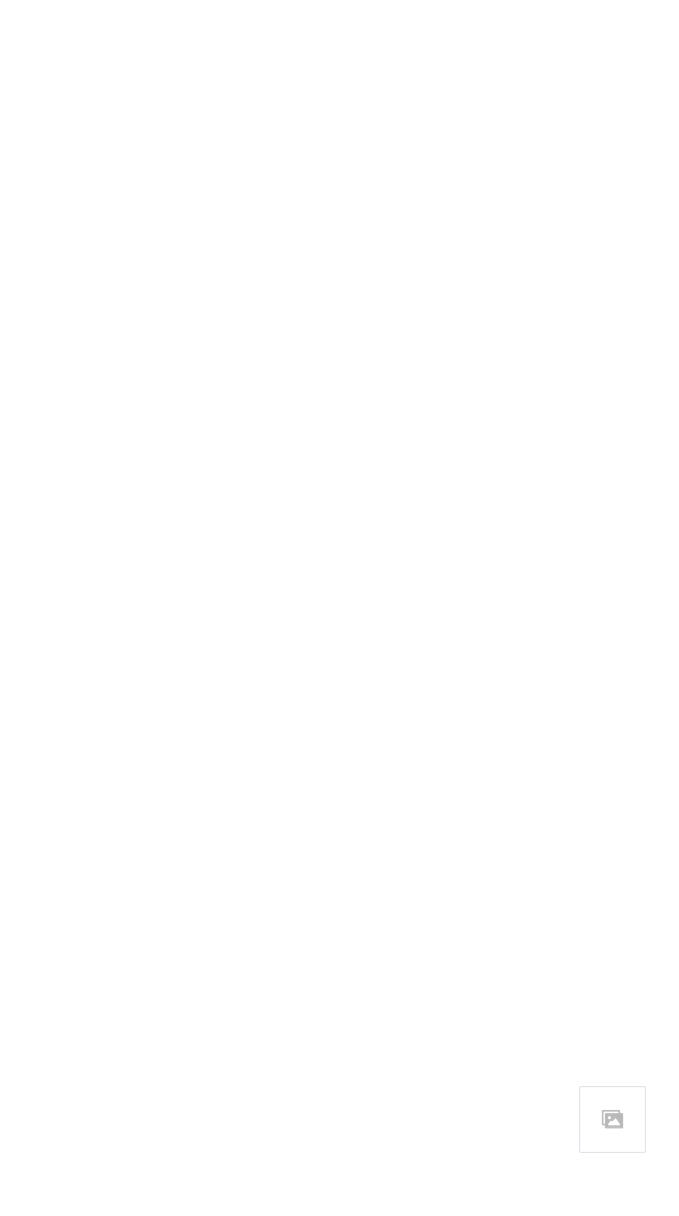This image depicts a small, gray-outlined square icon against a white background, representing a printer. The icon, typically found on toolbars for printing documents, portrays a detailed printer with a darker front section and an illustration of paper emerging from it, emphasizing its functionality. Measuring less than an inch, it symbolizes the familiar command used for printing tasks, often also triggered by the keyboard shortcut Ctrl+P.